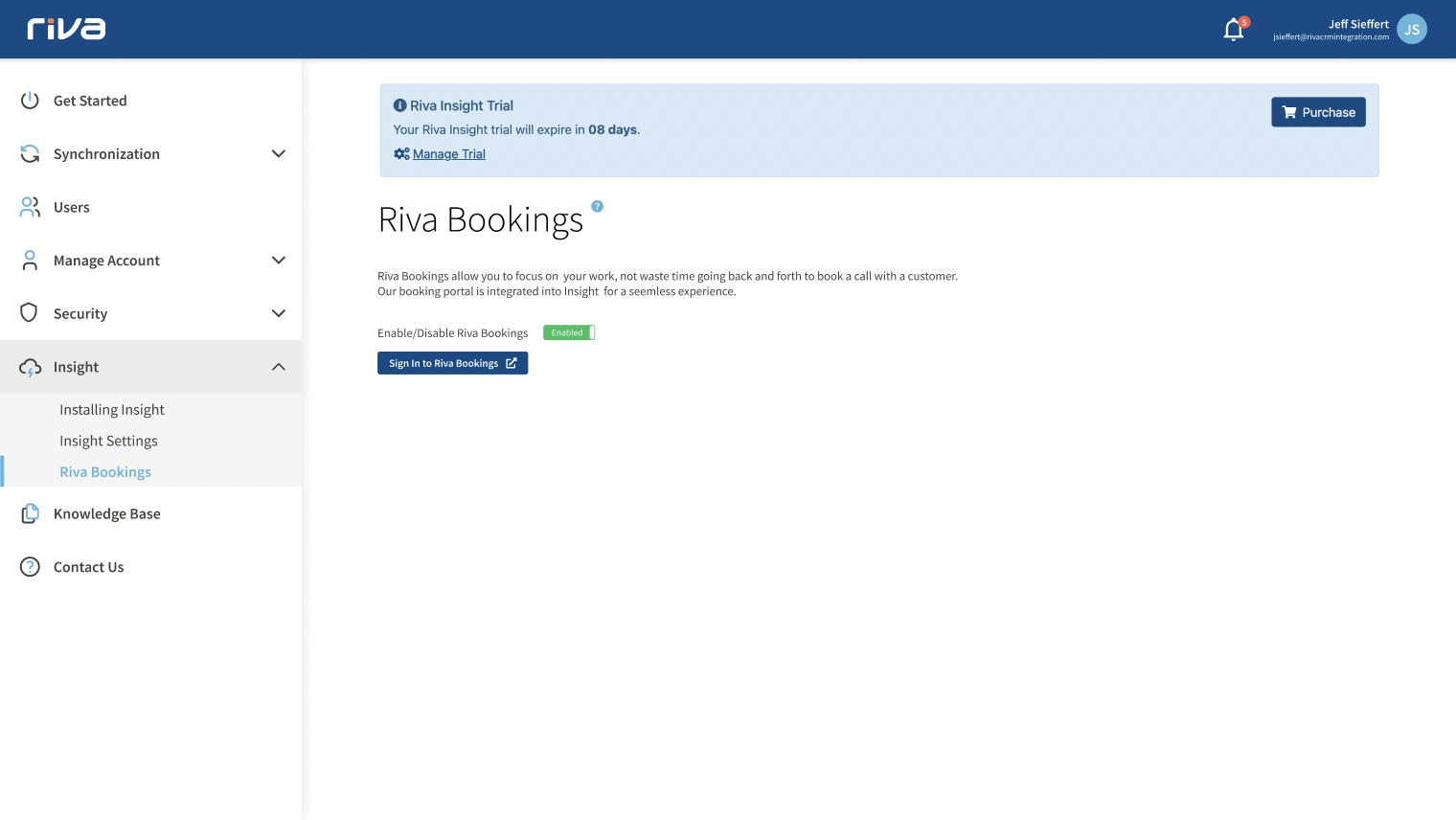The image depicts a website with a striking blue navigation bar at the top, prominently displaying the name "Riva" in bold, white letters. To the left on the bar, there is a notification icon resembling a small bell, indicating multiple alerts, though the specific count is unclear. Adjacent to this icon is the name "Jeff Seifert" next to a circular avatar containing the initials "JS."

On the left-hand side of the webpage, a vertical menu showcases various navigation tabs, organized as follows: "Get Started," "Synchronization," "Users," "Manage Account," "Security," "Insight," "Knowledge Base," and "Contact Us" at the bottom. The "Insight" tab is expanded, revealing subtabs labeled "Installing Insight," "Insight Settings," and "Riva Bookings," suggesting active user engagement with the Insight features.

Dominating the center of the webpage is the "Riva Bookings" section, alongside a clear notification about the "Riva Insight Trial," which will expire in eight days. Options to manage the trial and a shopping cart button labeled "Purchase" are prominently displayed. Below this, explanatory text reads: "Riva Bookings allows you to focus on your work, not waste time going back and forth to book a call with a customer. Our booking portal is integrated into Insight for a seamless experience." Two interactive options, "Enable" and "Disable" Riva Bookings, offer further customization.

This comprehensive layout suggests a user interface designed to streamline workflow and enhance user experience, focusing on practical functionality and ease of navigation.